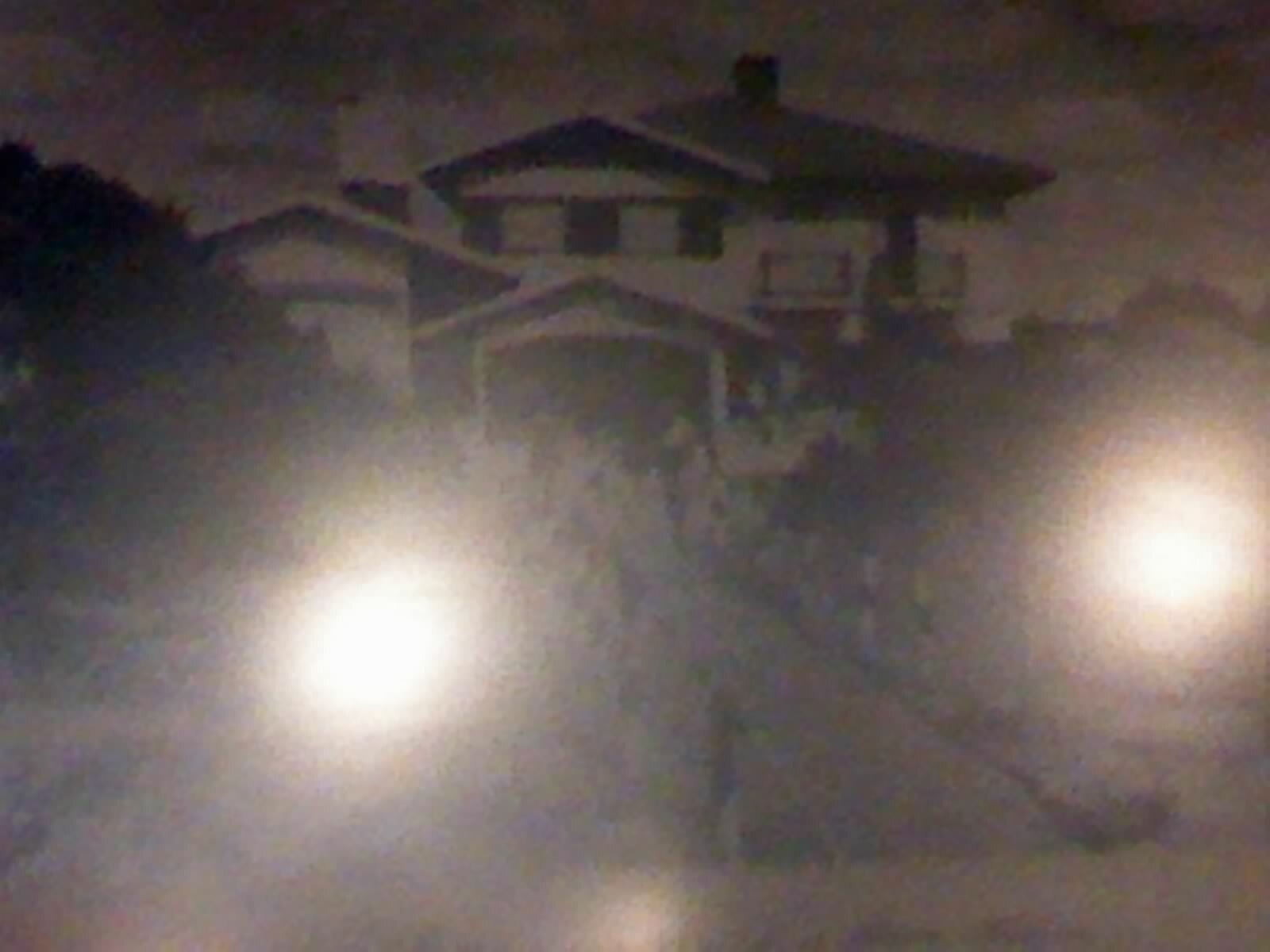This black and white photograph captures a large two-story house at the center, framed by two noticeable light reflections on either side that obscure the edges of the image. The prominent walkway, lined with flowers or plants, leads directly up to the house, creating a welcoming path. To the left of the walkway stands a substantial tree with a canopy of branches and leaves extending toward the right, providing a natural frame.

The house itself is painted white and adorned with darker colored shutters on the upper floor, adding a contrasting touch to the facade. Two small Juliet balconies are visible on the right side of the house, with the right-hand door open to the balcony and the left-hand door closed.

The entryway features an angular roof, matching the angular architectural style seen throughout the house, including the second-floor roof and the presumed garage roof to the left of the porch. The home's rooftop is punctuated by two chimneys: one situated on the left and the other prominently centered high on the roof. This detailed depiction offers a glimpse into the stately and picturesque setting of the residence.